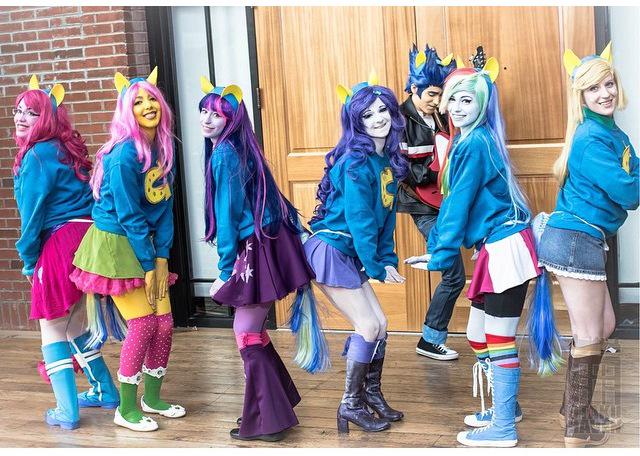The image depicts a lively and colorful scene at what appears to be a convention or costume meetup. Six high school-aged girls are the focus, each dressed in vibrant costumes inspired by My Little Pony characters. They are all wearing matching blue plush turtleneck sweaters adorned with a yellow horseshoe emblem. Their skirts, tights, socks, and shoes are in various bright colors such as pink, green, yellow, and blue, creating a rainbow-like effect. Each girl sports a headband with yellow donkey ears and wears a differently colored wig—blonde, blue, purple, indigo, pink, and red. Many of the girls have their faces painted to match their outfits, enhancing their playful and whimsical appearances.

In the background, partially obscured by the girls, stands a teenage boy with striking blue hair. He's dressed in blue jeans, black leather jacket with white and red stripes, and black Converse shoes. He also wears a headband with yellow ears, complementing the girls' accessories. The boy holds a guitar, adding to his rock-inspired look. This detailed and colorful ensemble suggests the group is participating in a My Little Pony-themed cosplay event, celebrating their favorite characters with elaborate and coordinated outfits.